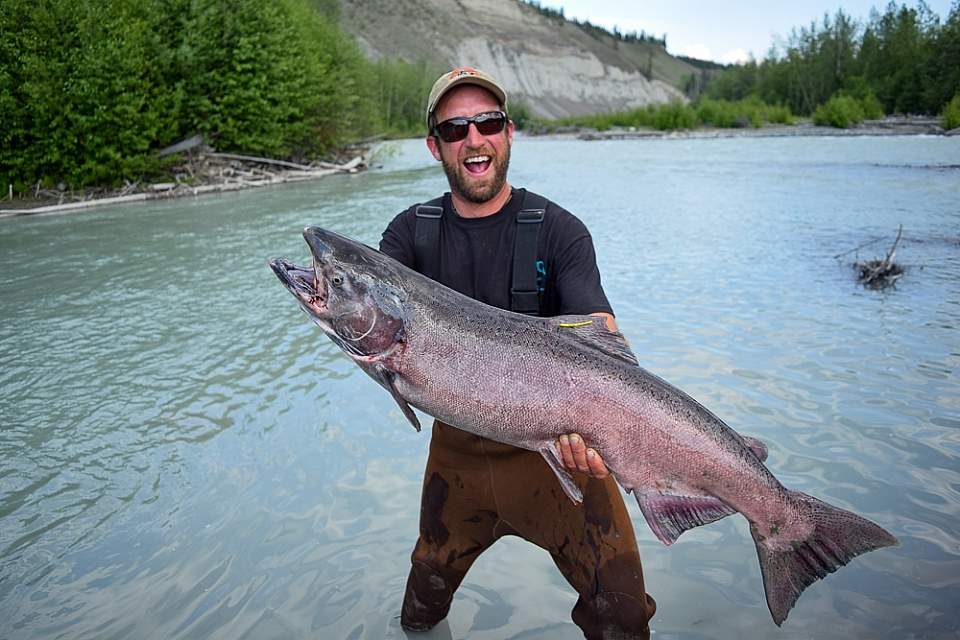In this vivid portrait, a man stands triumphantly in the middle of a river, smiling widely with his mouth open, showcasing straight, white teeth. His short-sleeved black T-shirt and brown waders, with visible straps over his shoulders, hint at a successful fishing expedition. He sports sunglasses and a light-colored, possibly yellowish baseball cap, partially concealing his short beard. The centerpiece of his achievement is a massive fish, likely a salmon or steelhead, which he holds with both hands—one under its midsection, the other supporting its head. The fish, tagged on its upper fin, has its mouth open, mirroring the man's exuberant expression. Surrounding him, the river's murky waters suggest glacial origins, and in the background, a landscape unfolds: sandbanks descend to the river's edge, cluttered with driftwood and debris, while trees flank both sides. A gravel bar with low shrubs is visible behind him, with larger trees further up and a glimpse of blue sky peeking through. The distant mountains appear barren and gray, contrasting with the lush greenery and capturing the serene, rugged charm of this natural fishing haven.